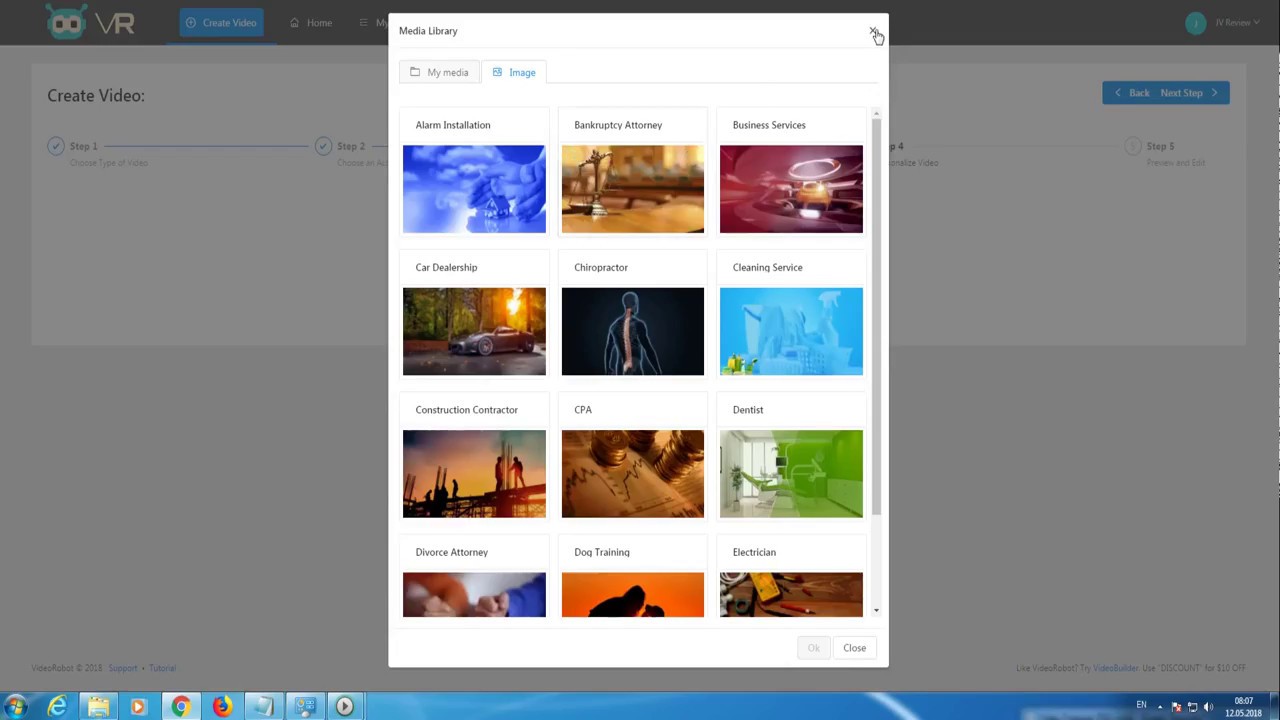This image is a screenshot of a web page. The main focus is a vertical, white rectangle window centered on the screen, titled "Media Library" at the top left corner. Below the title are two tabs: "My Media" (which is closed) and "Image" (which is open and highlighted in blue). 

Inside this window, there is a grid layout displaying a total of twelve images, though only nine are fully visible while the bottom three are partially cut off. Each image is framed in a rectangle and represents various categories. 

The first image in the top left corner is labeled "Alarm Installation" and features a mostly blue scene with a blue sky and clouds. A person’s hand is cupping a tiny house on a shiny platform, casting shadows. 

The second image is labeled "Bankruptcy Attorney," showcasing a scales of justice. 

The third image, titled "Business Services," follows, though its specific visual content isn’t fully described. 

Next is "Car Dealership," which includes a car. 

"Chiropractor" displays a person’s back with emphasis on the spine. 

"Cleaning Services" shows a collection of cleaning supplies. 

"Construction Contractor," "CPA," "Dentist," "Divorce Attorney," "Dog Training," and "Electrician" or "Election" (with visual content not specified) images follow in the sequence. 

At the bottom of the window are two actionable buttons labeled "OK" and "Close."